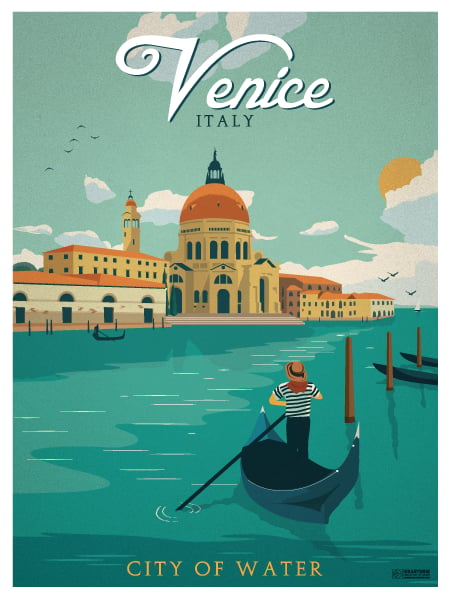The vertically aligned rectangular image resembles a magazine cover with a predominantly green background, including a green-shaded sky adorned with white and gray clouds. At the top, the text reads "Venice" in white letters, followed underneath by "Italy" in all caps with a smaller green font. The centerpiece is an imposing domed building featuring a middle dome with rectangular extensions on either side, primarily orange and brown in color with some white and yellow details. The foreground displays a dark green body of water with light green highlights and dashed white lines suggesting ripples.

On the lower right, a man is sitting and rowing a blue, pointy boat with white tips. The man, visible from the back, wears a brown hat, a black-and-white striped short-sleeved shirt, black pants, and a red scarf or orange bandana around his neck. The scene includes black birds flying in the sky to the left, with the sun visible on the right, accompanied by more birds below the clouds. Additional boats and poles are suggestive of a docking area, contributing to the scene's authenticity. At the bottom, in all caps and light brown letters, the text reads "City of Water."